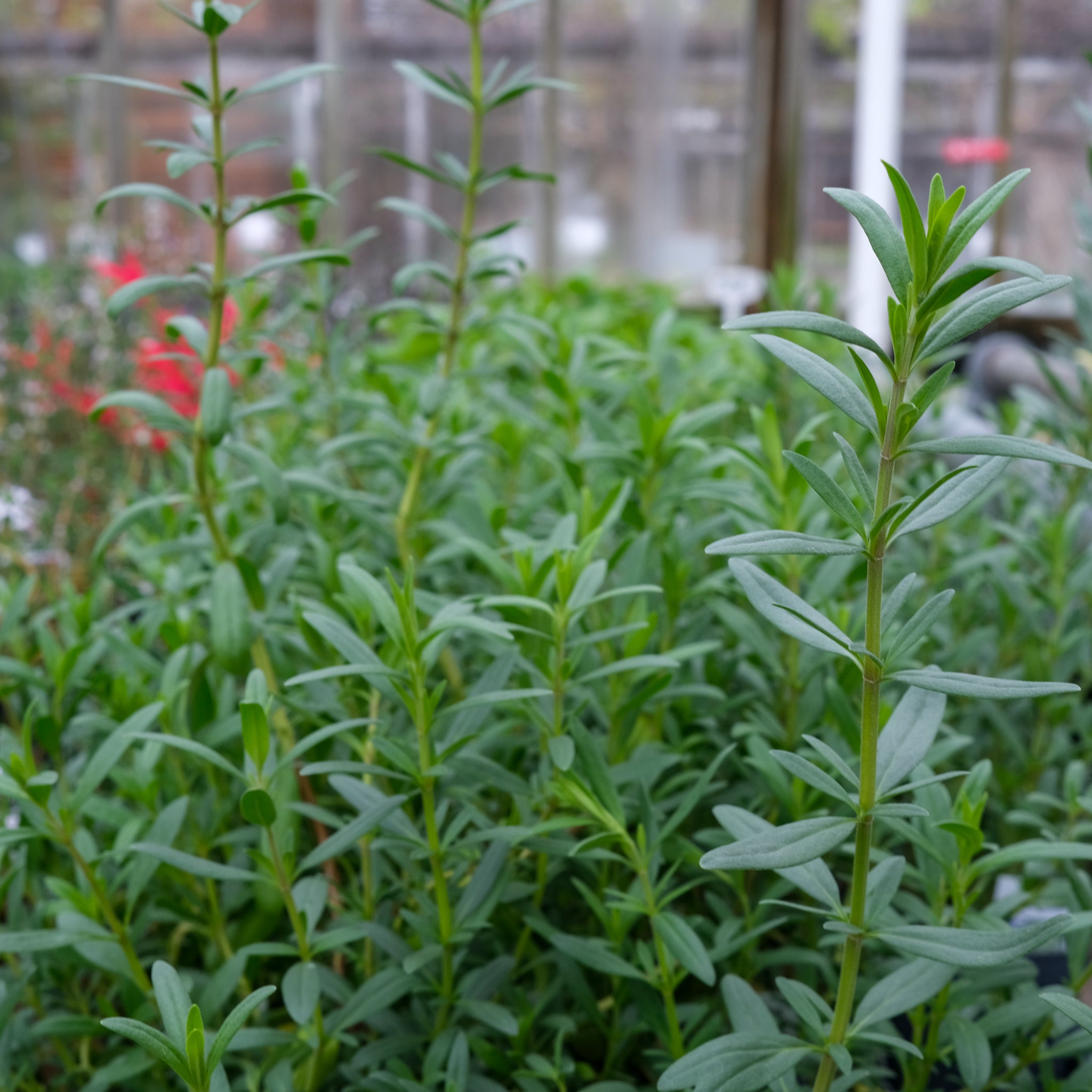This photograph captures a close-up view of numerous green plants, each featuring long, yellowish-green stems and narrow leaves sprouting uniformly from them. The strong depth of field effect emphasizes a single plant in sharp focus on the left side, while the rest blur into the background. This background includes indistinguishable elements of red, white, brown, and gray, hinting at potential buildings, a white pole, and garden-like structures, suggesting an outdoor urban setting possibly within a city park. Despite the blurriness of the backdrop, the lighting is adequate, lending decent detail to the plants. The uniformity and vertical growth of the plants make it difficult to identify their specific type, and notably, there are no flowers, buds, animals, people, or text present in the image.